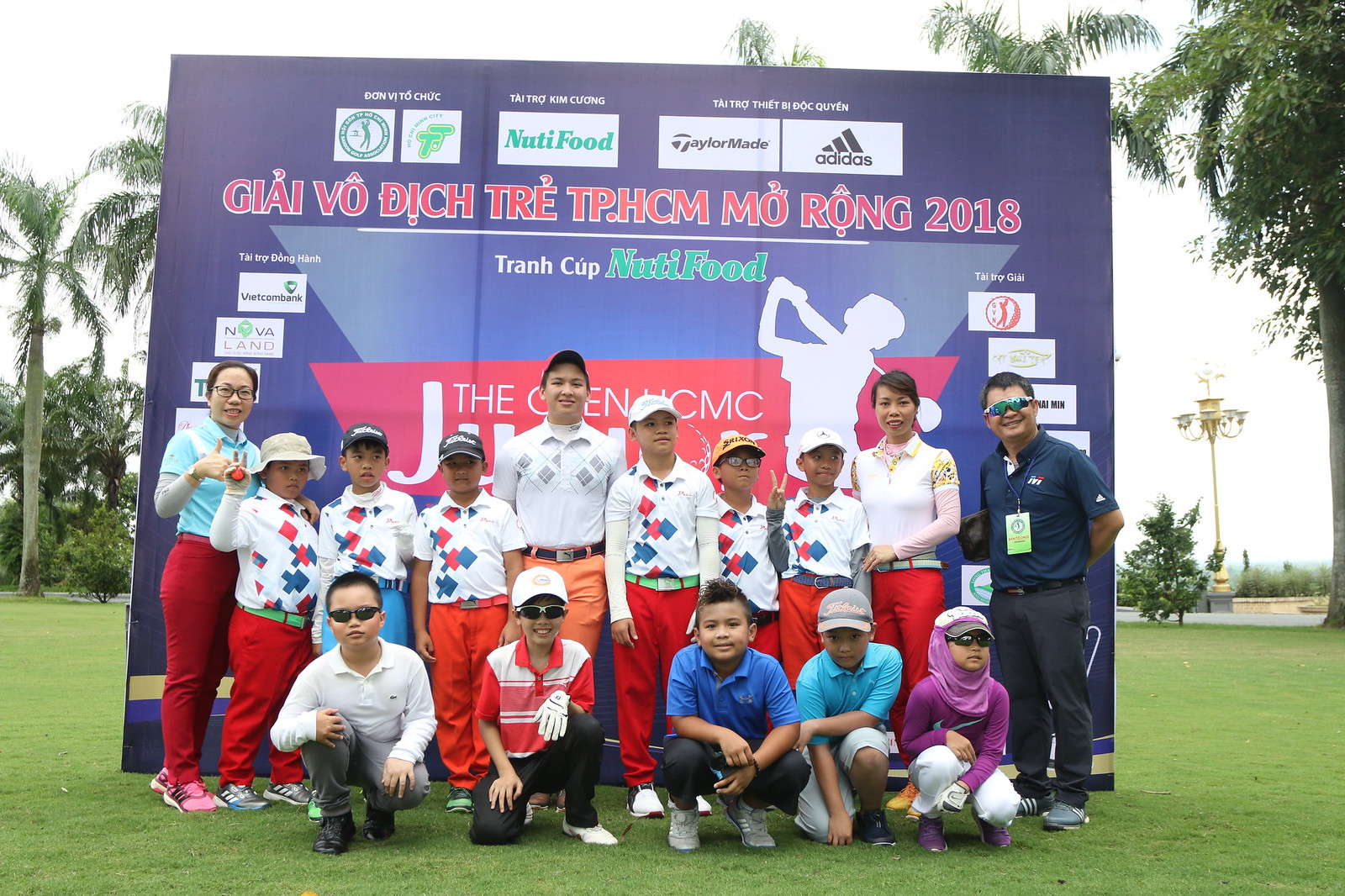This outdoor image captures a group of children and a few adults assembled in front of a large purple sign, set against a backdrop of palm trees and a clear blue sky. The sign features various sponsors, including NutriFood, TaylorMade, and Adidas, along with text that appears to be in Vietnamese, likely reading "GIAI VO DICH TRE TPHCM MỞ RỘNG 2018", suggesting an event related to a golf tournament. The group consists of about ten boys, with some standing and others kneeling on a grassy area. Many of the children are wearing ball caps and sunglasses, with varied colors such as blue and white. Among them, two boys in the front have sunglasses, and the one on the end has a scarf, sunglasses, and a ball cap. The adults are dispersed among the children, with everyone arranged neatly for the photograph.